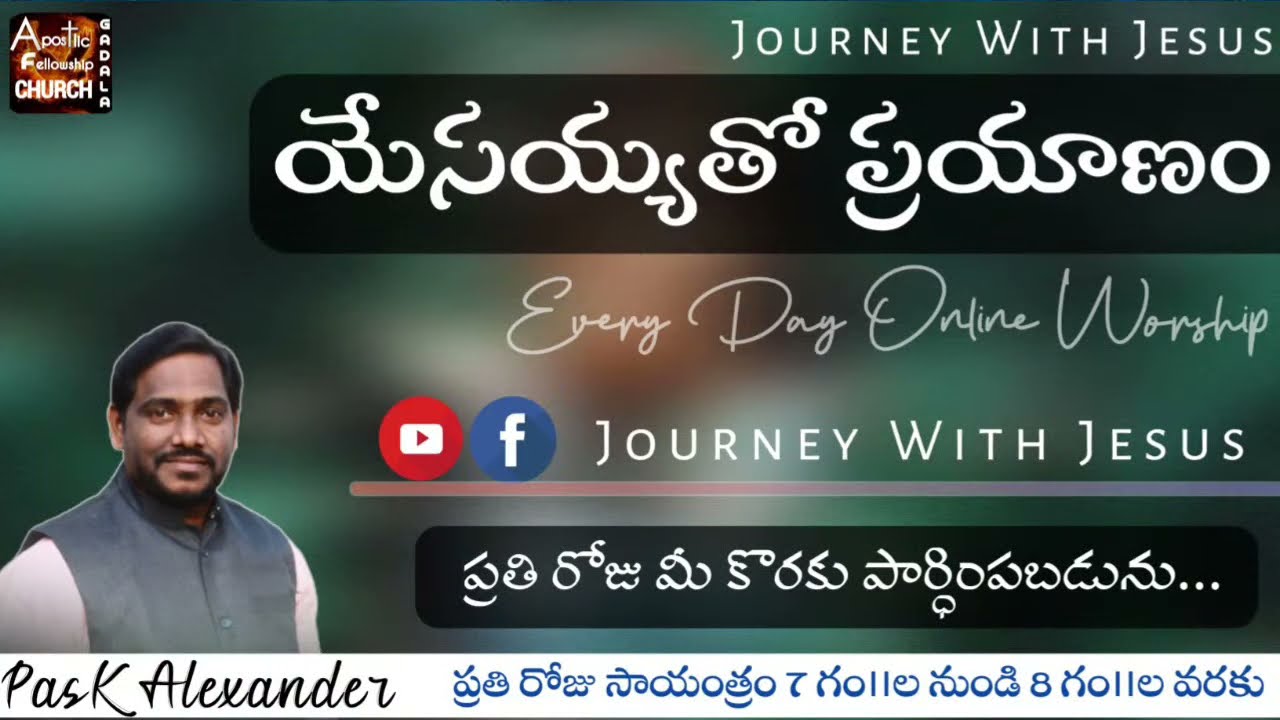The image is of a web page, possibly for a religious online workshop. The background features a blurry, green design with various pieces of information in English and another language, possibly Middle Eastern. At the top center, it reads "Journey with Jesus" in white text, followed by the same phrase in another language. Below, it says "Everyday Online Worship." Near the top left, the text "Apostolic Fellowship Church" is visible.

In the bottom left corner of the image, there's a picture of a man named Pasch K. Alexander, identifiable from the text nearby. He is smiling, wearing a gray vest over a white shirt, with a neatly trimmed beard and mustache, and dark hair combed to the side. The page also includes icons for YouTube and Facebook, suggesting links to these social media platforms.